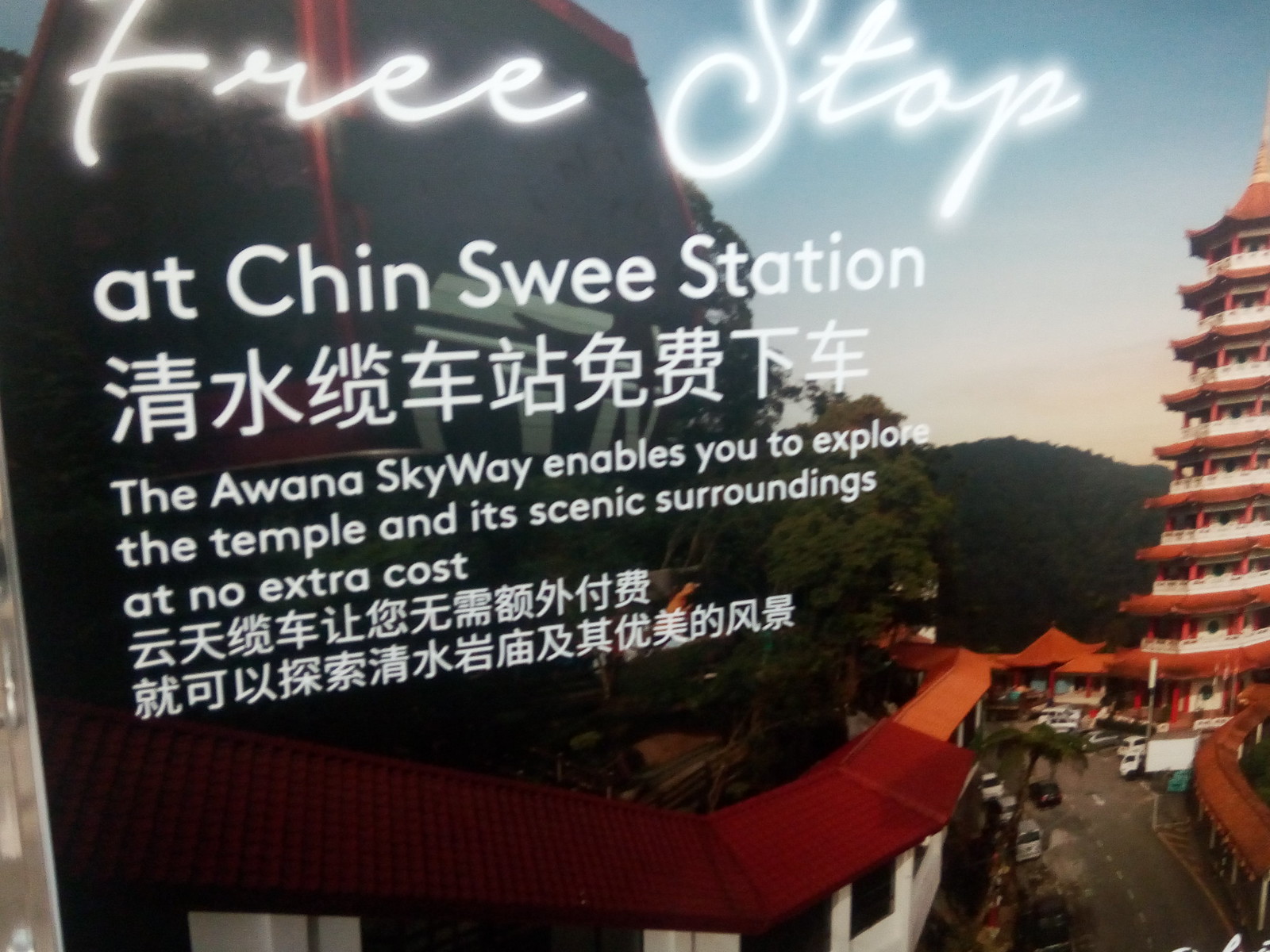The advertisement showcases a picturesque scene dominated by a traditional-looking Asian temple. This high-rise, multi-tiered building features a distinct oriental design, characterized by red and white colors—with red roofs and possibly white balconies or railings on each of its several floors. The temple, which appears to have eight or nine levels, includes a pointed, red-tiled roof at the top. Surrounding the temple are other architectural structures with red roofs and white exteriors, set against the backdrop of a lush green, mountainous hill.

In the foreground, there is a street with a visible parking lot and several small cars. The overall landscape suggests a scenic and serene setting, further embellished by the tall trees scattered throughout the background. 

Across the top of the image, in a cursive white font, it reads "Free Stop at Chinsui Station," accompanied by some Chinese characters. Beneath that text, the advertisement highlights, "The Oana Skyway enables you to explore the temple and its scenic surroundings at no extra cost," with additional Chinese text following. This composition effectively conveys a vibrant, cultural, and accessible tourist destination.